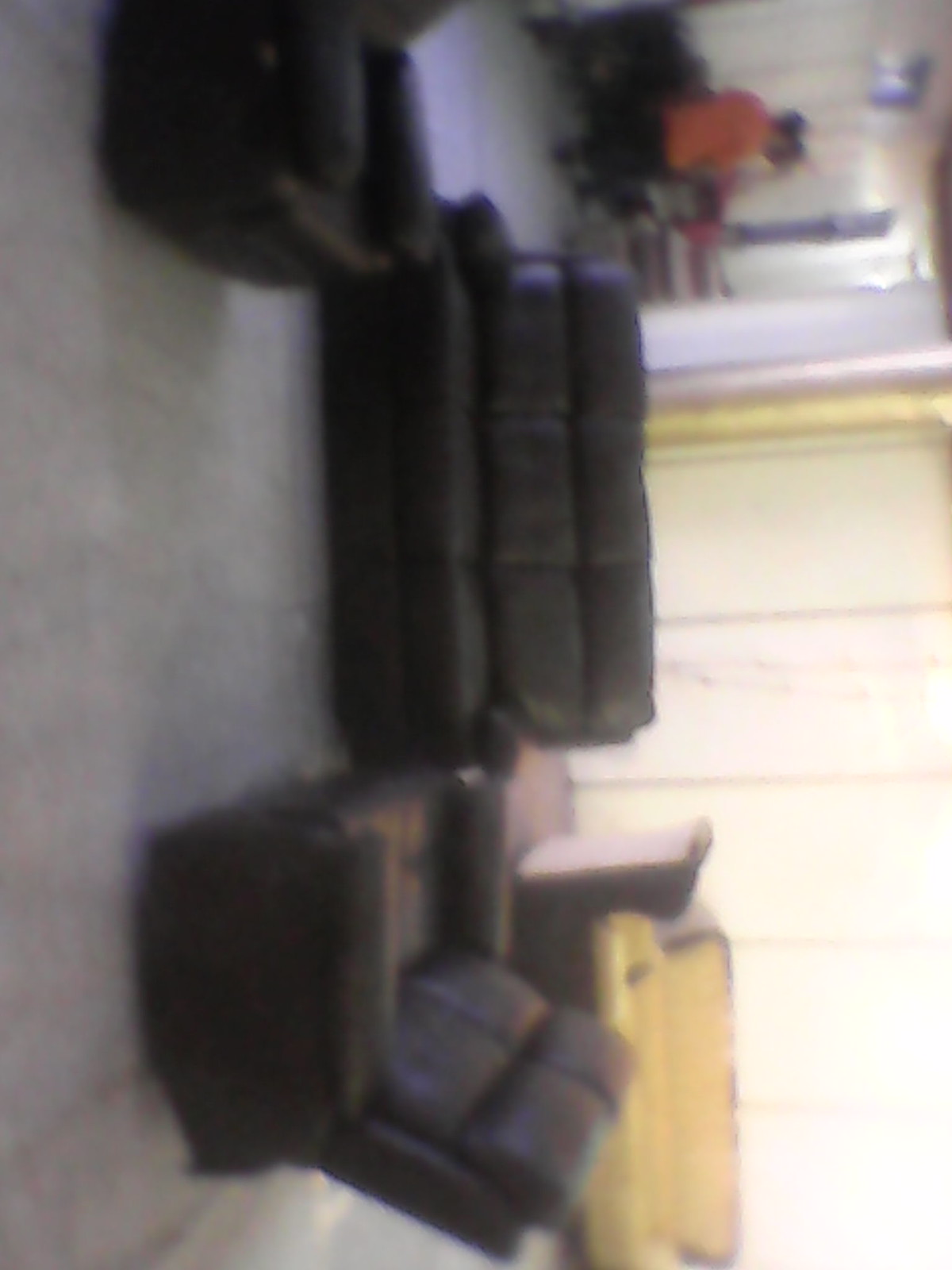This image, rotated 90 degrees to the right, depicts a living room set characterized by black furniture. At the center of the composition are three black leather couches, each adorned with black cushions and featuring square designs on the backrests. Visually aligned to the right due to the rotation, the couches seem to be leaning. Towards what would be the bottom right in its usual orientation, there's another piece of furniture with black and yellow elements, likely a couch with a yellow cushion.

The room itself, although blurry and slightly out of focus, reveals additional details. In the background, a person wearing a red t-shirt and black trousers appears upside down due to the image's rotation, standing near a white door frame. The flooring looks like laminate and the walls are painted white, with a possible window area covered up in the distance. The overall lighting suggests a significant amount of natural light entering the room.